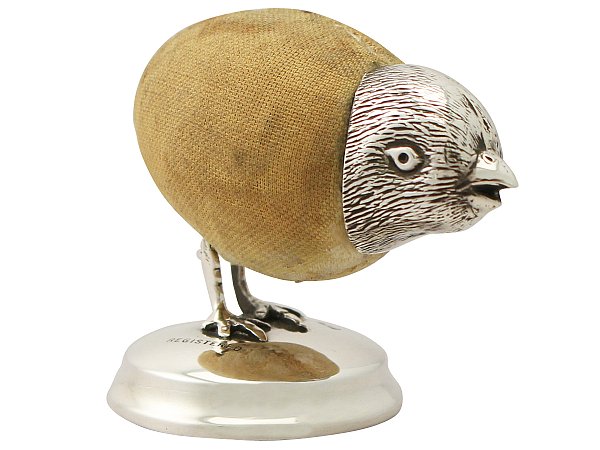This close-up image showcases an intricate bird figurine standing against a plain white background. The bird's head, beak slightly open, and legs, down to the detailed toes, are all crafted from silver, with one bead-like eye adding a touch of realism to the head. Its round, egg-shaped body is covered in a burlap material, providing an interesting texture contrast to the polished silver. The figurine stands on a silver base, which features an engraving, though the inscription is unclear. Notably, the bird lacks tail feathers and wings, leaving a simplistic yet captivating sculpture comprised only of its head, body, and legs.